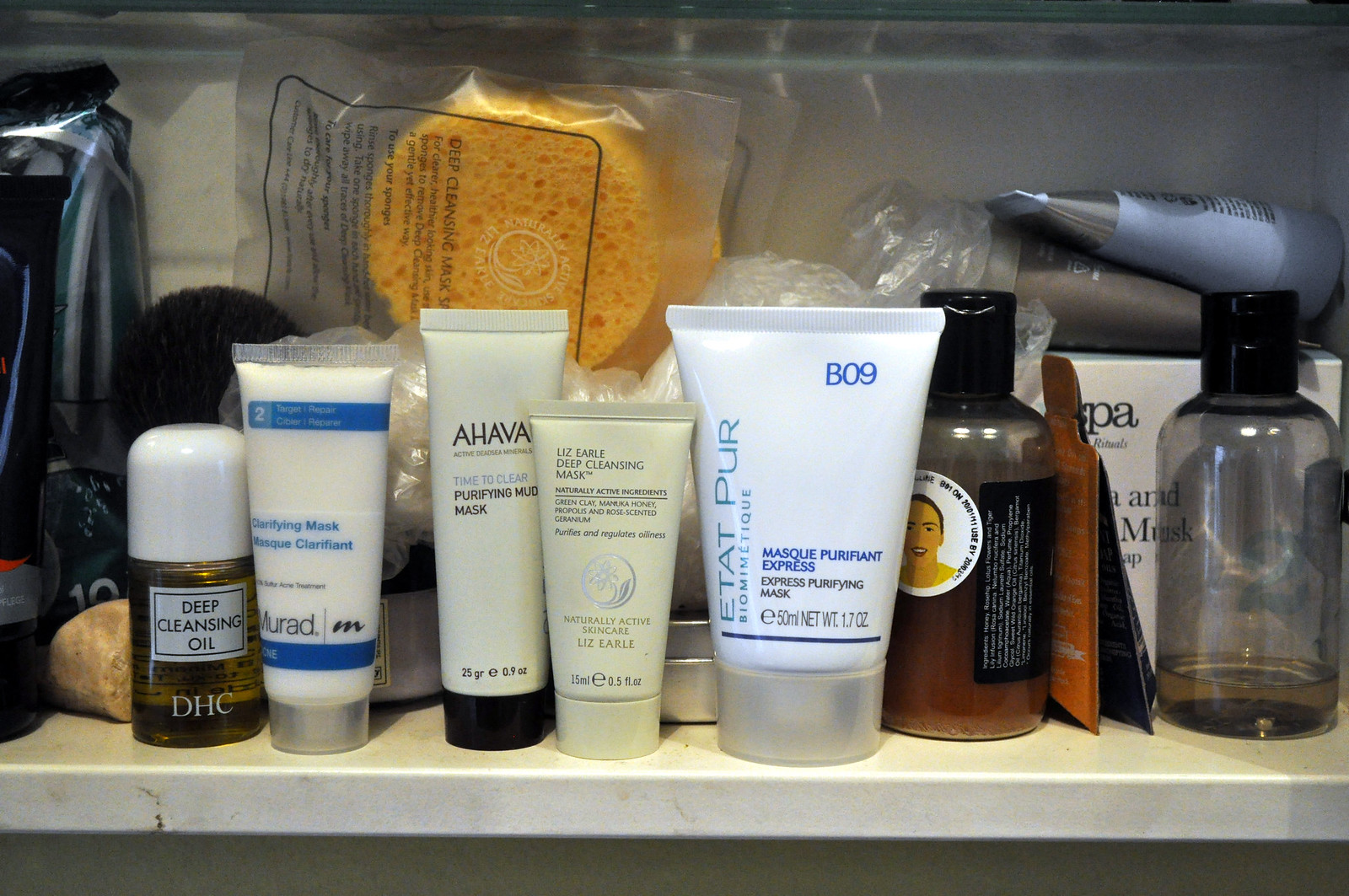The image depicts the lower shelf of a bathroom cabinet, meticulously arranged with a variety of personal care products. The shelf itself appears to be made of white stone or a marbled material, with gentle, darker squiggled lines creating a subtle, elegant pattern.

From left to right, the shelf houses an assortment of bottles and containers. The first item on the left is a clear cylindrical bottle with a white cap, featuring a label that prominently reads "Deep Cleansing Oil" in black text on a white background, and below in smaller white text on the clear bottle itself, it says "DHC", filled with a yellowish liquid.

Next, there are four plastic, tube-like bottles standing upside down with their lids facing downward. These containers have a design reminiscent of toothpaste tubes, tapering at the end where they are sealed.

To the right of these tubes is a larger cylindrical bottle adorned with a white sticker illustrating a cartoon face of a woman. The text on the label is not legible, and the bottle is capped with a black top. Adjacent to it, there is another cylindrical bottle, this one a darker, clear hue, also capped with black.

Adding to the collection, behind these front-row bottles, is a yellow circular sponge encased in clear plastic wrap, sealed with a label featuring black printed text and a black rectangular border.

The assortment of bottles and containers, organized neatly on the shelf, showcases a variety of personal care essentials, each distinct in shape and design, providing a glimpse into the owner's daily grooming routine.